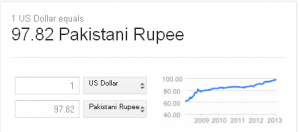The image provides a detailed snapshot of currency conversion between the U.S. dollar and the Pakistani rupee. It indicates that 1 U.S. dollar is equivalent to 97.82 Pakistani rupees. The interface features a box where users can input various currency values, supported by up and down arrows for easy navigation. Below this, another input field allows users to select the type of currency for conversion, showcasing U.S. dollar to Pakistani rupee in this instance. Users can presumably perform reverse calculations, such as converting 100 Pakistani rupees to U.S. dollars. Adjacent to these input fields is a historical graph illustrating the exchange rate trend from 2009 to 2013. Over this period, the exchange rate has shifted from approximately 80 to 97 Pakistani rupees per U.S. dollar, signifying a depreciation of the Pakistani rupee against the U.S. dollar.